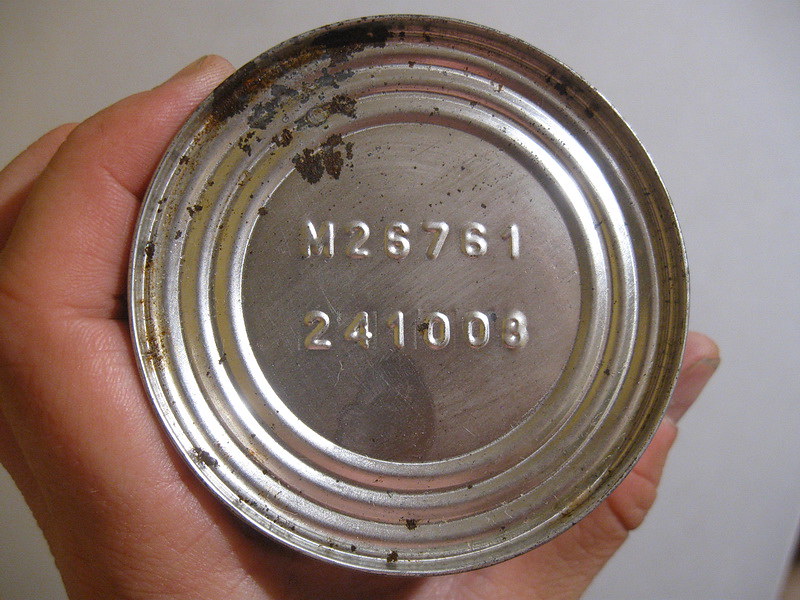A detailed photograph captures the bottom of an aluminum can, held upright by a person's hand. Only the round base of the can is visible, displaying its silver hue. The image highlights patches of rust that have discolored sections of the can, particularly noticeable as dark brown spots towards the upper corner. Imprinted on the silver surface is the text "M26761241008," which stands out against a small, contrasting white background.